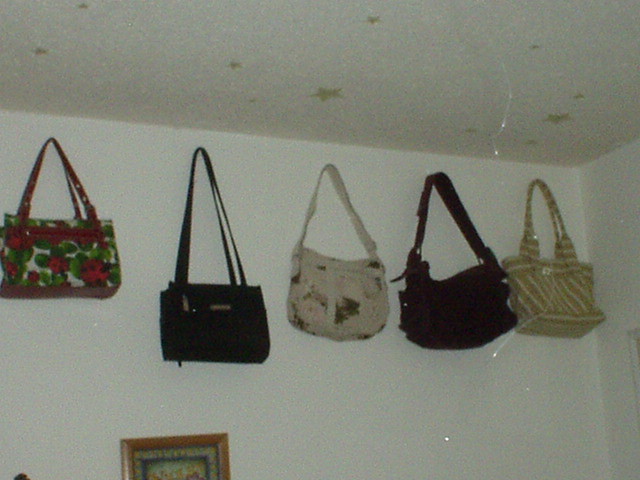This grainy, low-quality photograph depicts a corner of a white room, characterized by notable film grain and possible lens scratches. High up on the white wall, almost at the point where the wall meets the equally white ceiling, are five handbags hanging, their handles stretched out as though suspended by invisible nails. The ceiling features several glow-in-the-dark star decals scattered about.

Starting from the left, the first handbag is adorned with a print of ladybugs on green leaves, complemented by red handles. The second bag is entirely black with a long shoulder strap. The third handbag is a rounded, squat white bag with patterns too distorted to clearly discern but possibly floral. Moving to the fourth bag, it appears to be sportier, brown in color, with a wider strap and a lumpy shape, suggesting a utilitarian design. Finally, the fifth handbag features a design with yellow and white diagonal stripes, exuding a bright, cheerful aesthetic.

In the lower right corner of the photograph, the top of a wooden picture frame can be seen, although the contents within the frame remain indiscernible due to the image quality and lighting, which primarily seems to be from the camera flash.